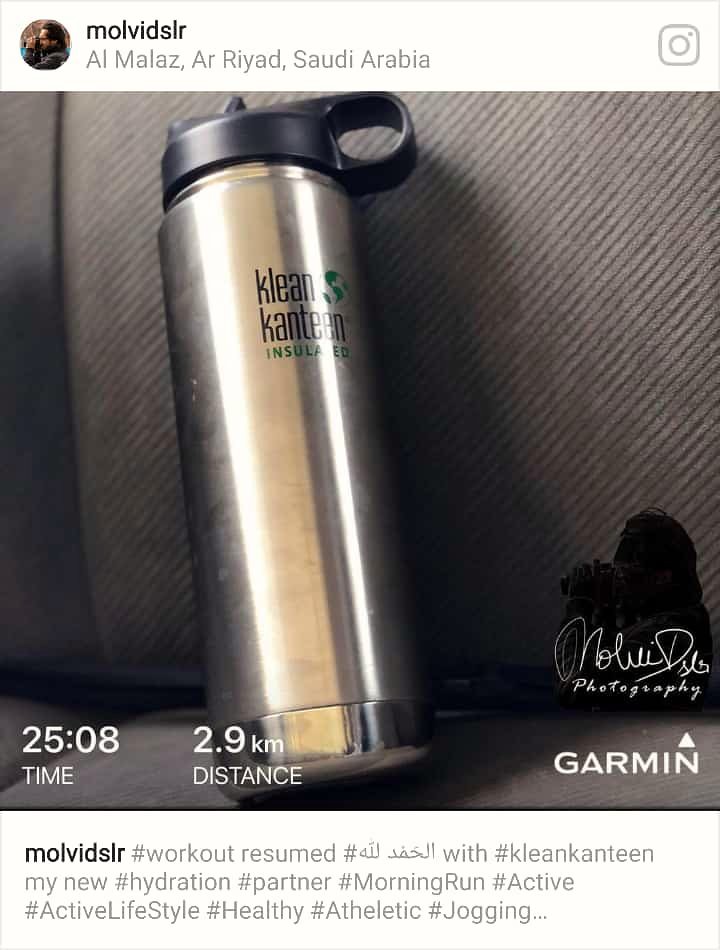This detailed Instagram post by user molvidslr, capturing an aluminum "Clean Canteen" insulated water bottle with a black lid, posed against a corduroy-textured, gray car seat, provides an inspiring snapshot of an active lifestyle. The water bottle features black lettering and a green globe insignia, symbolizing an eco-conscious choice. The post is geo-tagged to Al-Malaz, Riyadh, Saudi Arabia, and includes a timestamp of 2508 time and a distance of 2.9 kilometers, highlighting a morning run. The bottom right corner of the photograph showcases a watermark stating "molvidslr photography" in script, along with the word "Garmin." The caption emphasizes fitness and health with hashtags like #WorkoutResumed, #MyNewHydrationPartner, #MorningRun, #ActiveLifestyle, #Healthy, and #Jogging, accompanied by some Arabic text. The border on the image's bottom frame contains three lines of faint print, reinforcing the athletic narrative.